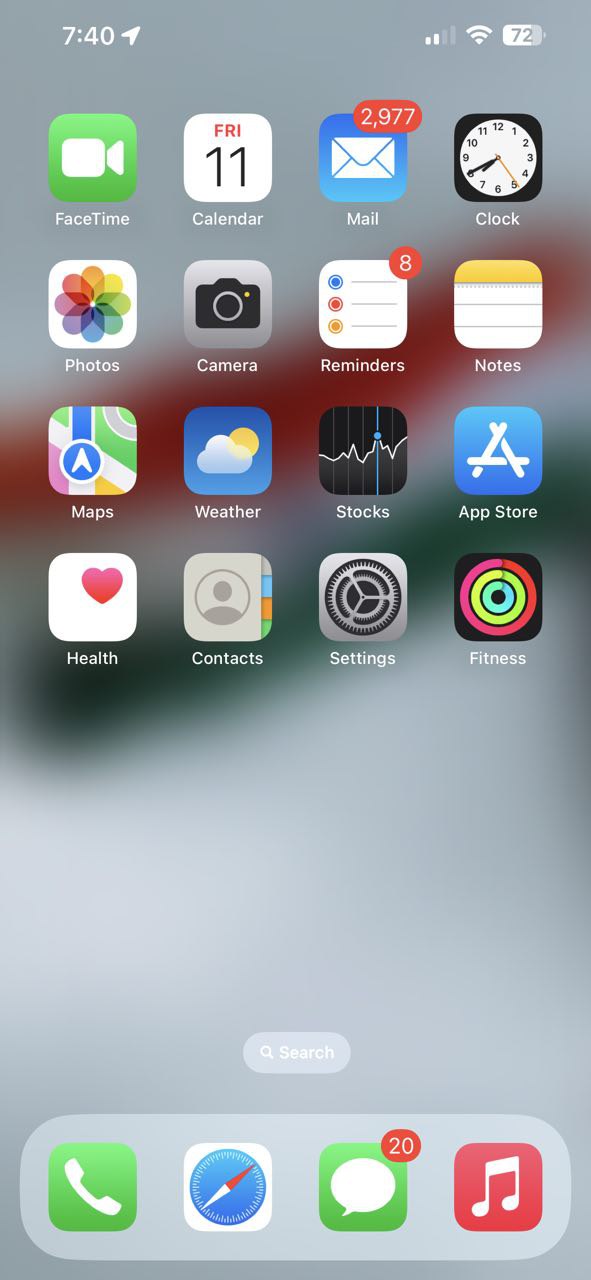The screenshot appears to be taken from an Android phone's home screen. The actual hardware of the phone is not visible, just the screen contents.

At the top left corner, the time is displayed as "7:40" accompanied by a diagonal upward-pointing arrow. To the right, there are signal indicators showing 2 out of 4 bars, followed by a fully-filled WiFi icon and a battery icon displaying "72%".

Beneath the status bar, several app icons are organized in a 4x4 grid. These include:
1. **FaceTime** - represented by a camera icon.
2. **Calendar** - showing "Friday the 11th".
3. **Mail** - depicted with an envelope icon and a notification badge displaying "2977".
4. **Clock** - symbolized by a clock icon.
5. **Photos**.
6. **Camera** - depicted by a camera icon.
7. **Reminders** - illustrated with an icon showing three bullet points.
8. **Notes**.
9. **Maps**.
10. **Weather**.
11. **Stocks**.
12. **App Store**.
13. **Health** - represented by a heart icon.
14. **Contacts**.
15. **Settings** - depicted with cogs.
16. **Fitness**.

Below the app grid, there is a small oval search button. Beneath that, there is a rectangular oval-shaped dock with four icons: Phone, Compass, Messaging, and Music.